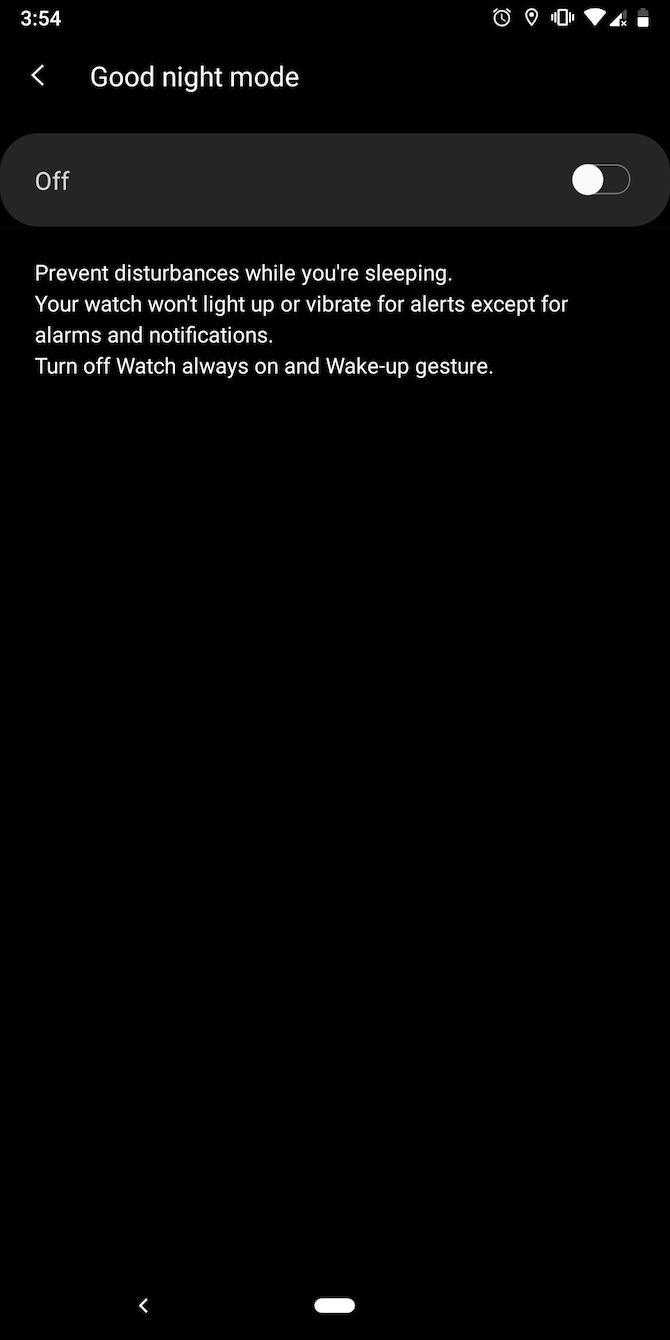The image appears to be a screenshot from a smartphone displaying the settings for "Good Night Mode." The primary feature, labeled "Good Night Mode," is toggled off, along with other related settings that are also in the off position. The description below explains, "Prevent disturbance while you’re sleeping. Your watch won’t light up or vibrate for alerts, except for alarms and notifications." Additional options include "Turn off watch always" and disabling the "wake up gesture."

At the bottom of the screen, there's a small circular button and an icon resembling a home page indicator. This screenshot primarily showcases the configuration options available to minimize distractions during sleep by controlling a wearable device's behavior.